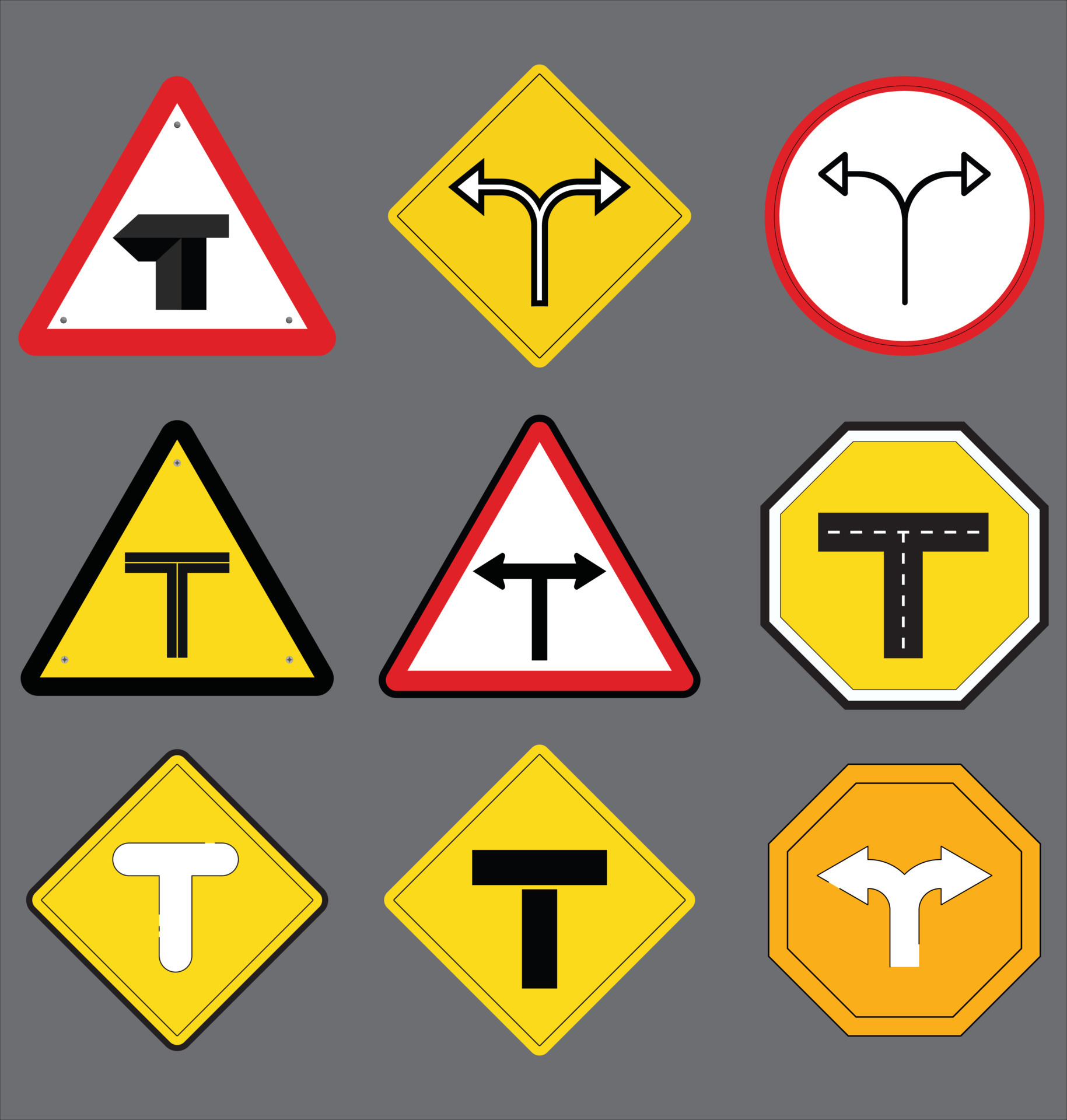This image is a square-shaped diagram with a grey background, featuring a 3x3 grid of 9 distinct traffic signs. Each sign illustrates different ways a street can dead-end, requiring a 90-degree turn either left or right. The signs are diverse in color and shape: 5 are yellow, 1 is orange, and 3 are white with red trim. The designs on the signs are primarily black and white. The shapes include 3 diamonds, 3 triangles with rounded edges, 2 octagons, and 1 circle. The images on the signs depict street layouts with the indication that one must turn left or right at the end of a street. The signs are unfamiliar, suggesting they may be used in a different country.